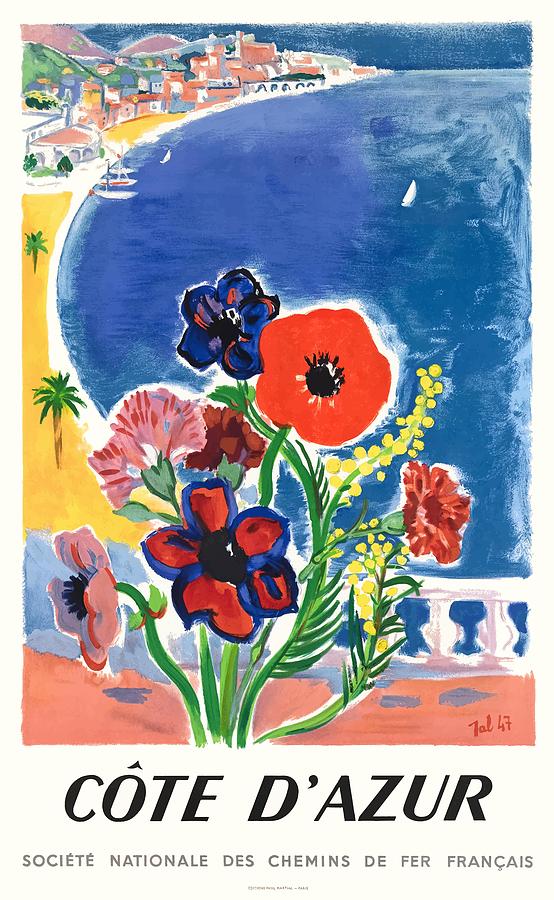This hand-painted image, labeled "TAL 47" at the bottom, depicts a vibrant and colorful coastal scene. Dominated by shades of blue, the painting features a towering mountain in the background with just a sliver of sky visible above it. To the left, pink hills frame the scene, leading towards a quaint village nestled along the shoreline. The village, characterized by its light orange and peach rooftops, sits behind a green hill. The white sandy beach connects to a stretch of yellow ground adorned with lush green palm trees.

In the foreground, a beautiful bouquet of red, blue, and pink flowers stands prominently, drawing the viewer's eye immediately. The calm blue water of the sea, likely the Mediterranean, stretches out from the shore with boats hitched to a dock, adding to the serene atmosphere. The bottom of the painting is inscribed with French text that reads "Côte d'Azur, Société Nationale des Chemins de fer Français," suggesting a picturesque location in France. This exquisite watercolor piece captures the essence of a coastal paradise, radiating vibrancy and tranquility.